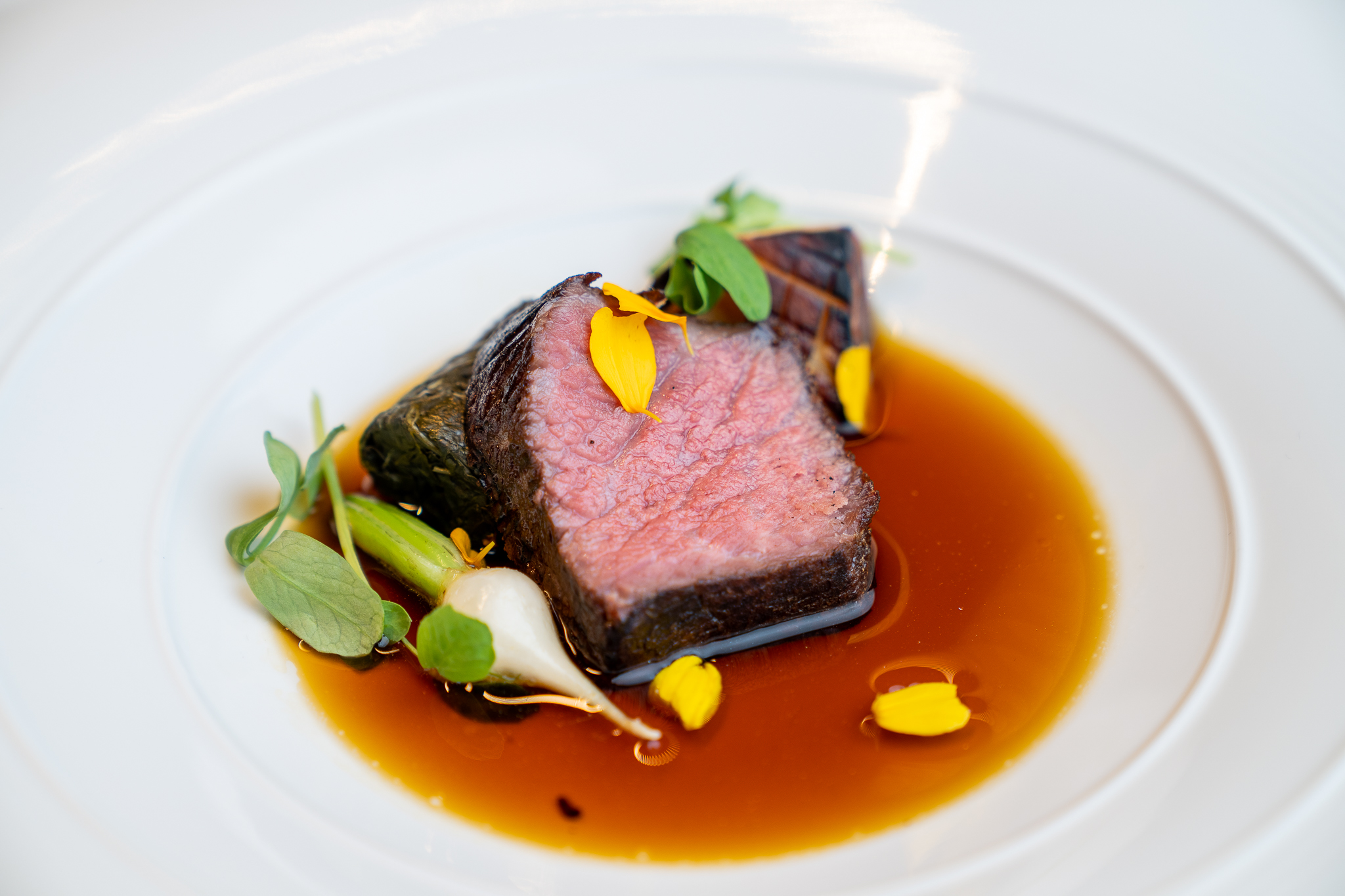The image showcases an elegantly presented dish, likely from a high-end restaurant or food website. At the center of a sophisticated white plate with subtle concentric circles that highlight its depth, several medium-rare slices of beef are displayed. The beef is cooked to perfection, with a beautifully browned exterior and a moist, pink interior. It is nestled in a delicate, amber-colored sauce that looks like a light broth. Adorning the dish are various aesthetic and possibly edible floral elements, including white and yellow petal-like additions. To the left and upper left of the main feature, there are some green garnishes and an unidentified plant with a green stem and a white bulb. All elements combined create a visually appealing gourmet presentation typical of upscale culinary art.